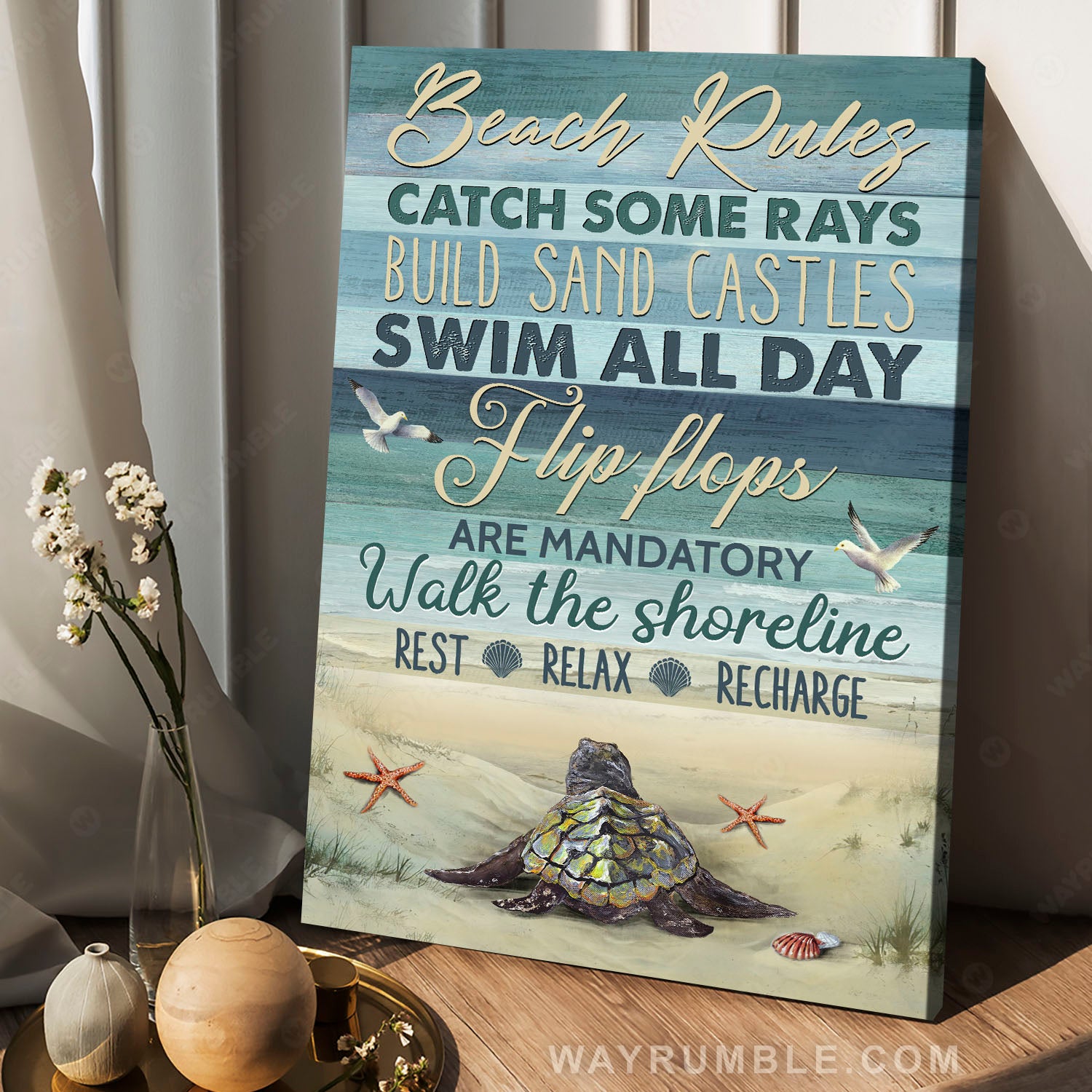The photograph captures a serene indoor scene featuring a small canvas picture leaning against a white wall on a light wooden desk or table. Sunlight filters through nearby open curtains, casting a warm glow on the setup. The canvas, highlighted by its blue and beige tones, depicts a beach-themed scene complete with a sea turtle, sand dollars, seashells, and a starfish against a backdrop of sand and ocean. Two seagulls soar above while green beach grass adds a touch of natural texture. The picture prominently displays the text "Beach Rules: Catch some rays, build sandcastles, swim all day, flip-flops are mandatory, walk the shoreline, rest, relax, recharge." To the left of the canvas, a vase filled with small white flowers sits on a gold, circular tray, alongside some spherical wooden objects. The overall composition is illuminated by the natural sunlight streaming in, creating an inviting and peaceful atmosphere.